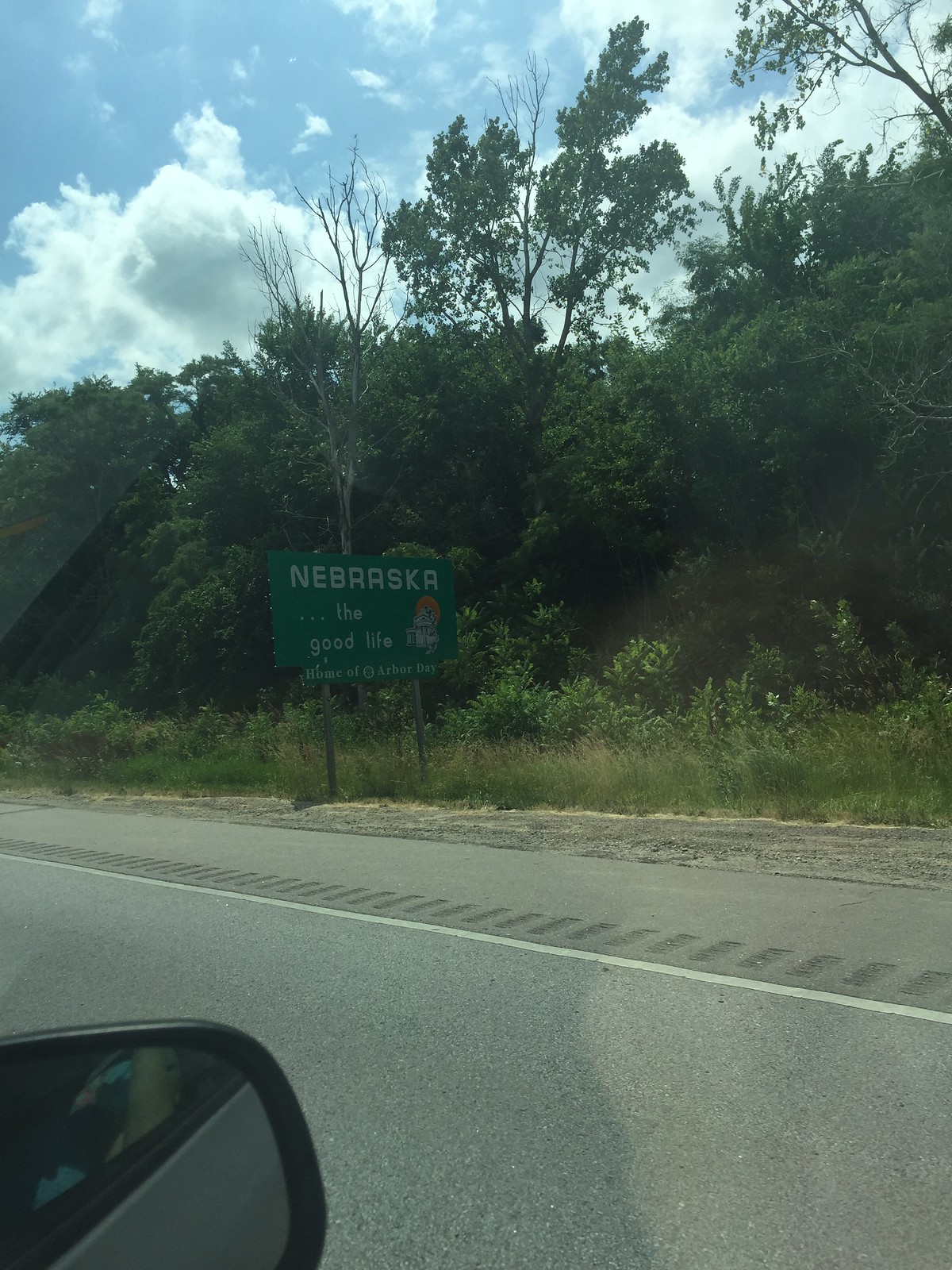A vibrant color photo taken from inside a car, likely from the passenger seat, captures a scenic view outside. Dominating the lower right corner, the rearview mirror hints at the vehicle’s presence. The open road, visible to the right, showcases a gray asphalt surface with a distinct white line painted on it, flanked by a dirt area.

Central to the image stands a prominent green street sign, emblazoned with the white text: "Nebraska ... The Good Life, Home of Arbor Day." Illustrations of tall trees, green bushes, and expansive, verdant grass surround the sign, weaving a lush tapestry of greenery. In the backdrop, a tall white house and a bright sun image underscore the sign's depiction of Nebraska's charm.

Above, the vast expanse of the sky is painted in a serene blue, dotted with large, feather-like white clouds that float leisurely, adding a sense of calm to the scene. The entirety of the image exudes a harmonious blend of natural elements, embodying the essence of "The Good Life" in Nebraska.